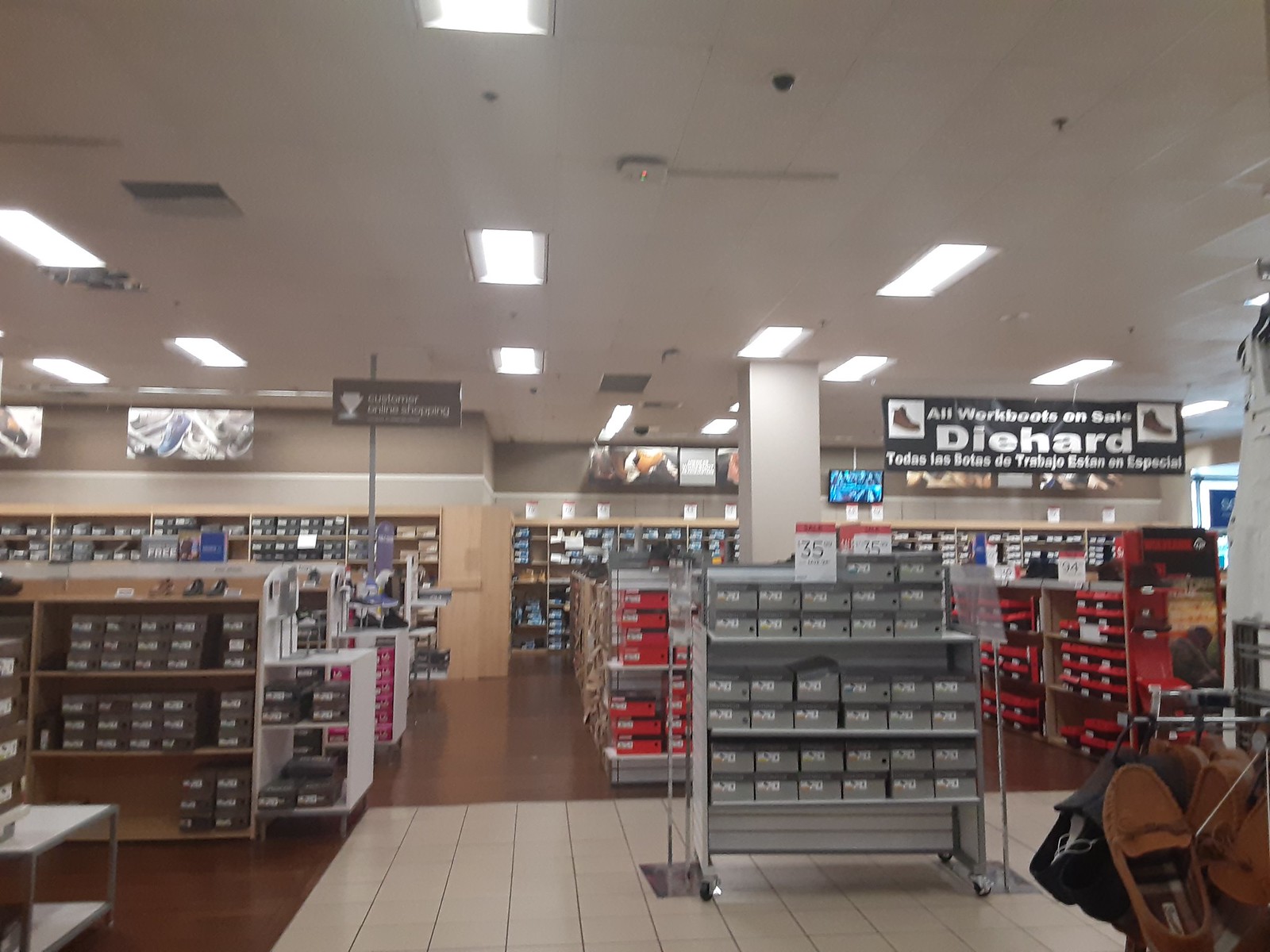The photo captures the interior of a bustling shoe store. The store is illuminated by multiple fluorescent lights on the ceiling, casting a bright light on the diverse array of footwear. In the far back of the store, a wooden display case is positioned against the hardwood floor, and rows of shelves align with boxes in red, white, and black. There is another shelf on the left side filled with gray boxes. In the center of the image, the flooring transitions from hardwood to white tiles, where a gray rack stands prominently, loaded with gray shoeboxes and a sign indicating a 35% discount. At the top right, a sign declares "All Work Boots on Sale," with additional text in Spanish underneath. To the bottom right, a rack brimming with brown leather loafers or moccasins can be seen. Scattered throughout the store, shoes are displayed on racks, shelves, and hanging from various stands, emphasizing the store's wide selection.